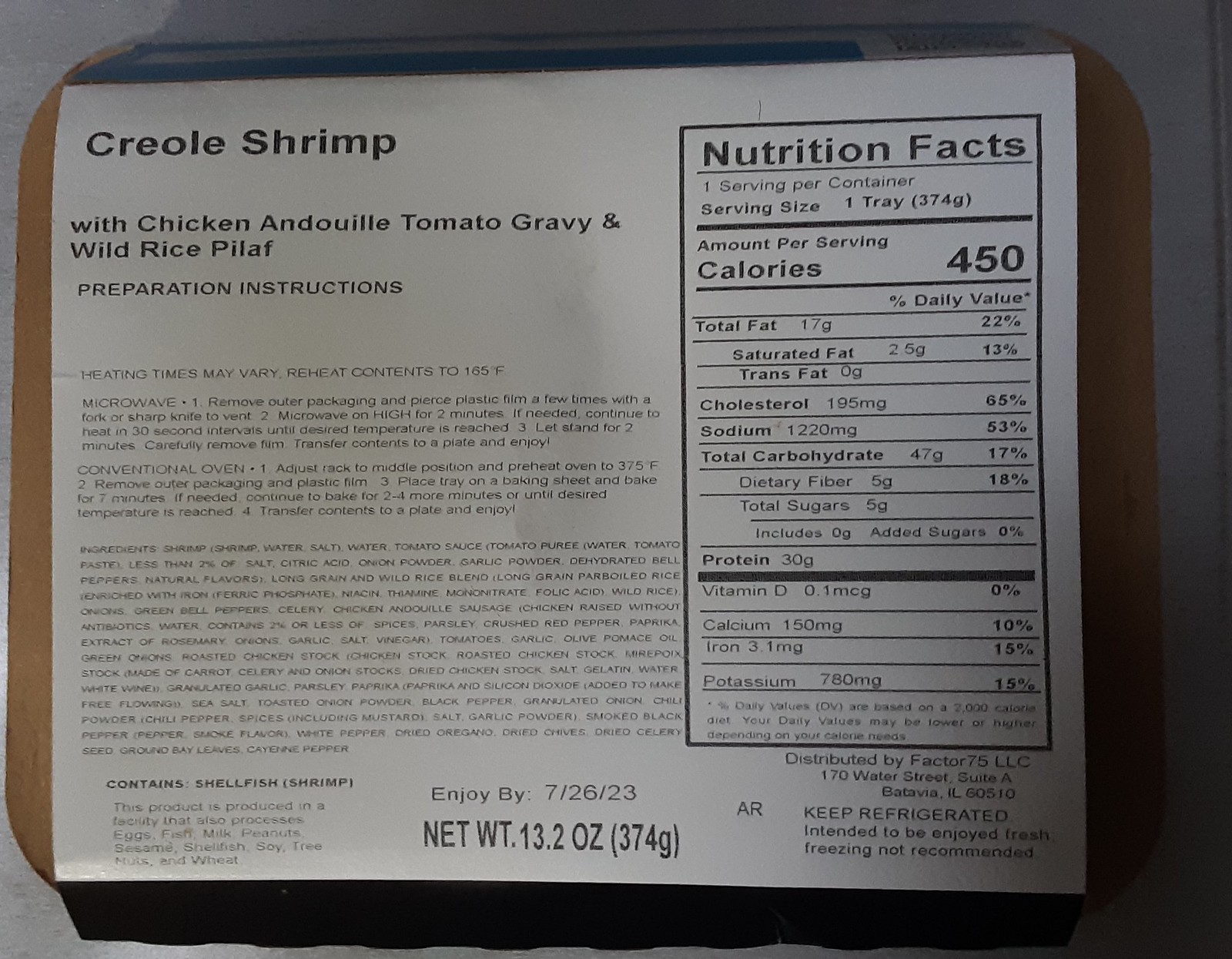A neatly packaged meal sits centered against a neutral gray background, accented by subtle brownish hues around the edges. Dominating the front of the package is a large, prominent white label adorned with clear black print. The label reads, "Creole Shrimp with Chicken Andouille, Tomato Gravy, and Wild Rice Pilaf," detailing the meal's enticing components. Below the title, a section contains the preparation instructions. A distinct black box with a white interior houses essential nutritional facts and serving sizes, indicating one tray at 450 calories. Additional nutritional information, including daily values, is meticulously laid out. At the bottom of the label, the net weight of 13.2 ounces (374 grams) is specified, along with a reminder to keep the product refrigerated until ready for cooking.